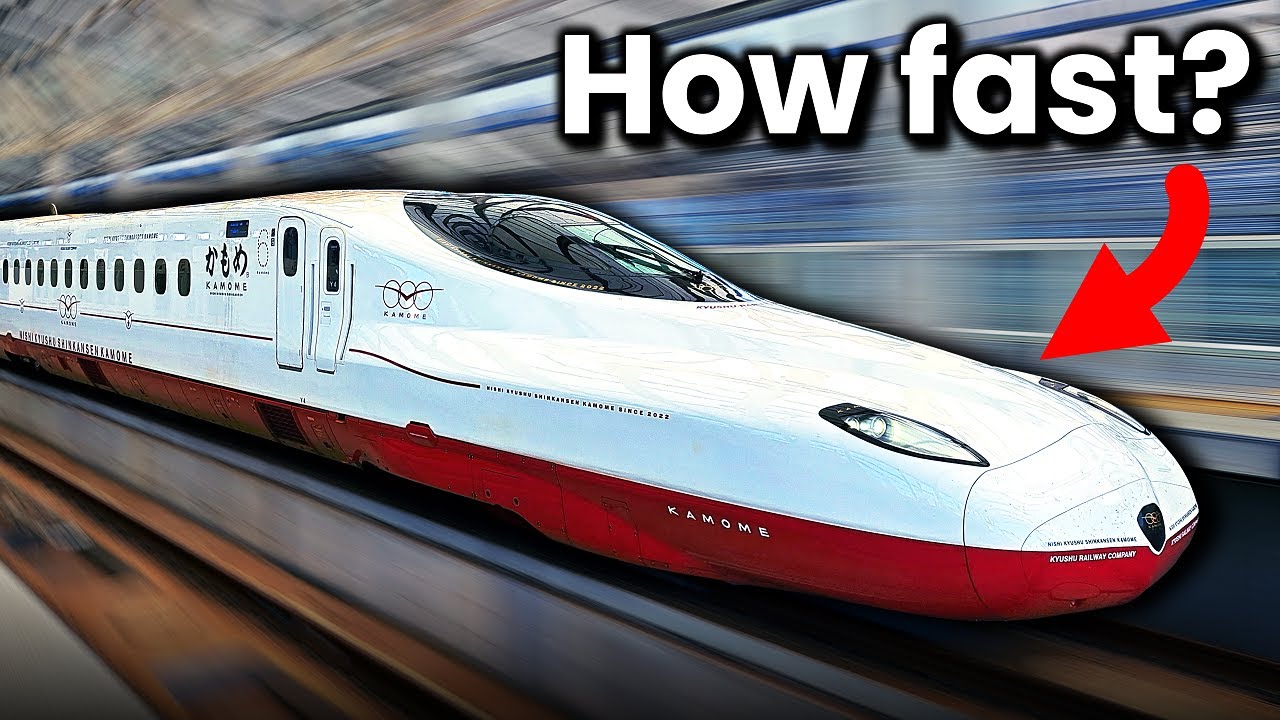The image features a centrally positioned, sleek bullet train named "Komome," with its nose pointed slightly to the right. The front and middle sections of the train are prominently displayed, showcasing a modern design with a white upper body, a red lower section, and black-tinted windows. The train, which has elements reminiscent of an airplane fuselage, sports two headlights and a contemporary windshield. Surrounding the train, the background is a blur of blues, grays, browns, and tans, indicating high speed and motion. At the top right of the image, bold white text with a black shadow asks, "How fast?" Below this text, a curved red arrow points directly to the train. The bottom left of the image features a blurred representation of the track the train is traveling on. The overall graphical style of the image emphasizes speed and movement, intending to provoke curiosity about the train's velocity.